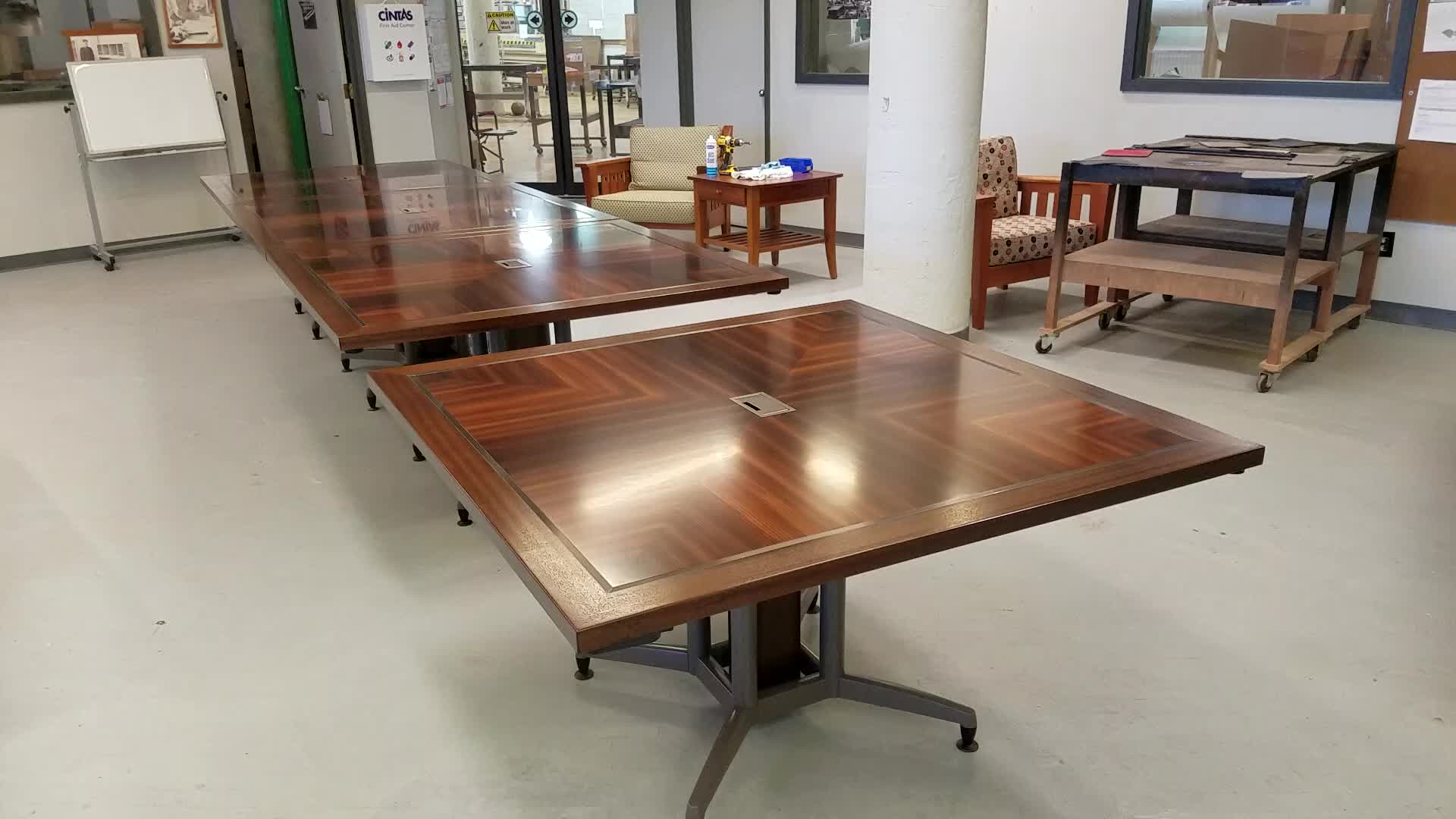The photograph captures an indoor furniture showroom featuring prominently two large, richly stained mahogany conference tables, supported by sleek metallic legs with rollers for easy mobility. The tables, polished to a bright shine, stand out against the white linoleum floor, enhancing their luxurious appearance. In the background, on the upper left, a whiteboard is visible, while to the right, several chairs, carts, and small desks complete the scene. A white pole is slightly right of center, adding to the structured layout of the room. This detailed setting suggests a sophisticated space designed for office or meeting room furnishings.